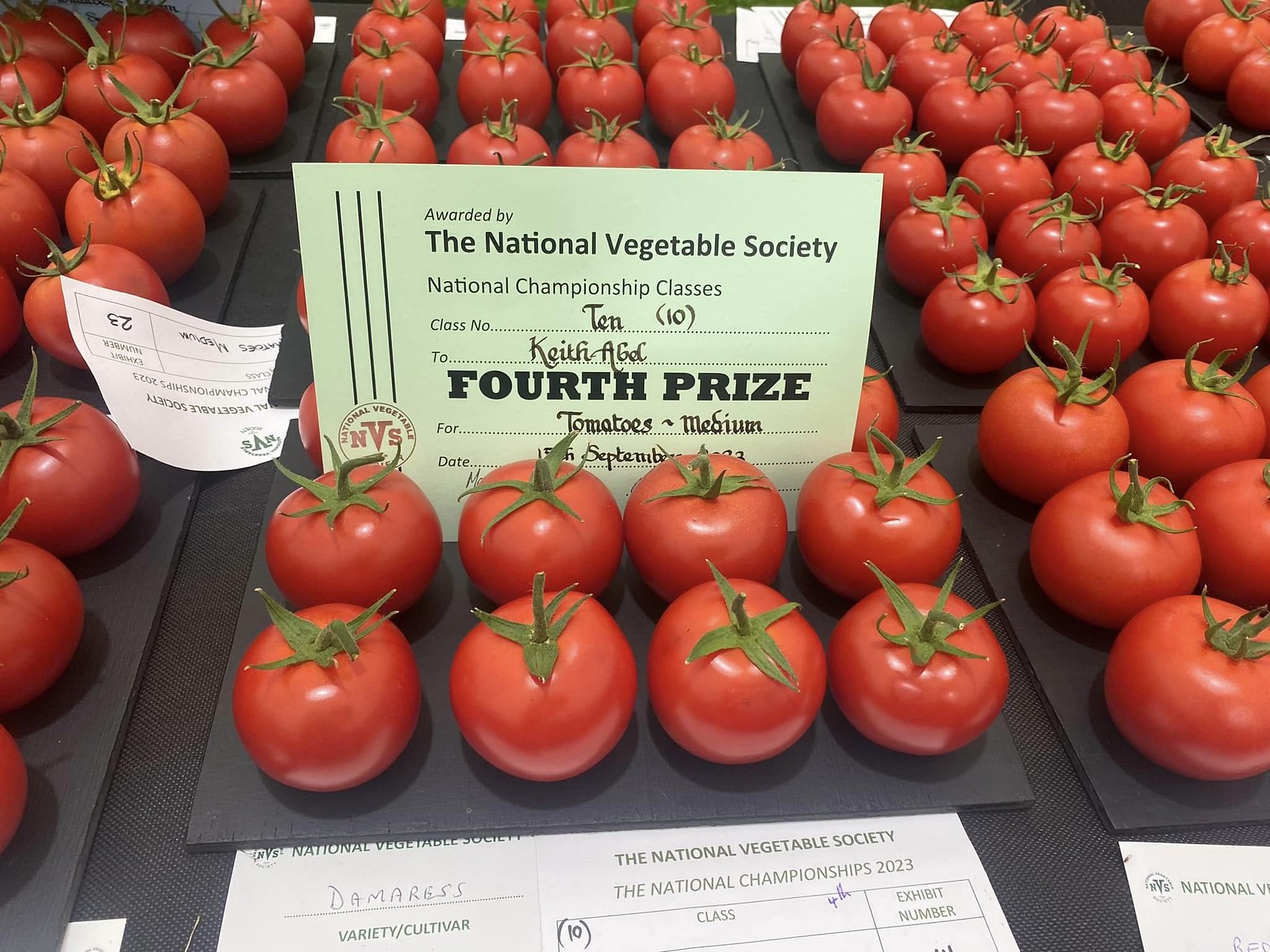The image showcases a bounty of perfectly round, red tomatoes with their little green stems intact, neatly arranged in rows on black cardboard surfaces. At the center of the tableau lies a certificate from the National Vegetable Society, awarded to Keith Abel for securing fourth prize in the National Championship Class Number 10 for medium-sized tomatoes. The certificate prominently features the words "awarded by the National Vegetable Society, National Championship Classes," and "fourth prize for tomatoes medium," though the full date is partially obscured with only "September" visible. Additionally, various other documents are scattered across the display, including a paper at the front that reads "National Vegetable Society, the National Championships 2023," and another piece mentioning the tomato variety "Damaris." The scene is a testament to meticulous cultivation and presentation, celebrating the accomplishment of an exemplary gardener.